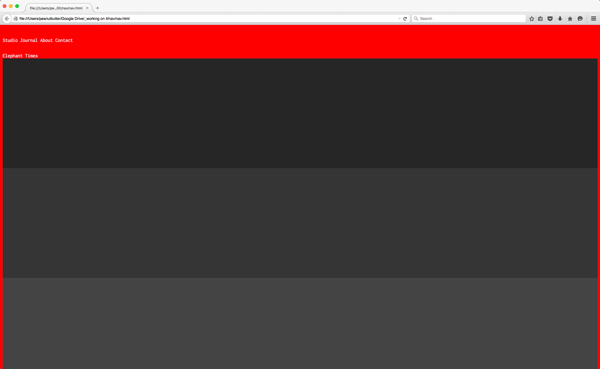The image features a simple yet detailed design set against a gradient gray background. At the top, there are geometric elements including a small green circle, red circle, yellow circle, and blue circle. Adjacent to these is another grouping of red, yellow, and green circles. 

Just below this section is a gray tab on a matching gray background, rendering it nearly unreadable. Underneath the tab is a recognizable back arrow icon, along with an unclear website address. A white search bar with the word "Search" in gray text is positioned below, alongside a row of icons: a star, briefcase, shield, down arrow, an unidentifiable symbol, a smiley face, and a trio of dots.

The inner section of the image contrasts with a bold red background and white text at the top reading "Studio," "Journal," "About," and "Contact." Below this header, text that appears to say "Elephant Times" or "Allegiant Times" is somewhat obscured and difficult to decipher.

The lower portion of the picture includes a dark gray bar, transitioning into medium and dark black bars, ending in a lighter gray bar at the bottom. The layout is clean and minimalistic, providing a straightforward visual hierarchy and a sense of structure without additional embellishments.